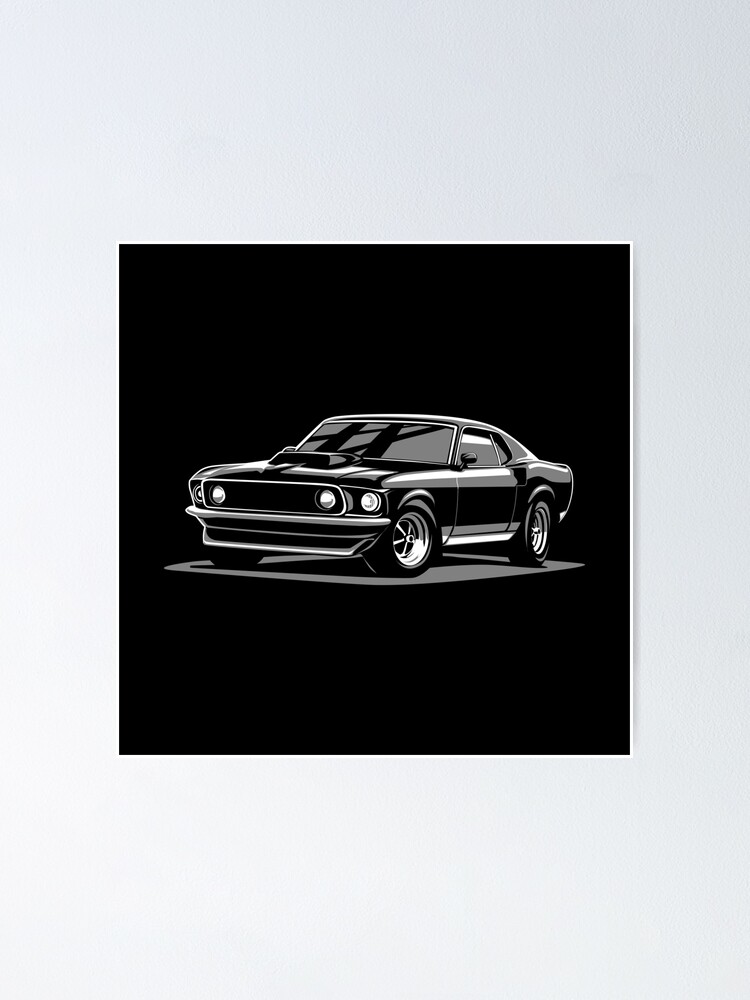This black and white image, which appears to be either digitally created or hand-drawn, features a vintage Ford Mustang muscle car set against a stark black background with a gray, off-white border. The Mustang, depicted in jet black, is rendered at a semi-angle, showing both the front from the left and a partial side view. The front of the car is characterized by a square body design, a hood with an air intake scoop, and four headlights. The car is further accentuated by its thick, deep dish rims and tinted windows. Underneath the car is a gray surface, and the black front grille adds to the vintage aesthetic. Despite being mostly monochromatic with black, gray, and white hues, the drawing skillfully captures reflections on the front windshield, contributing to its realistic feel.